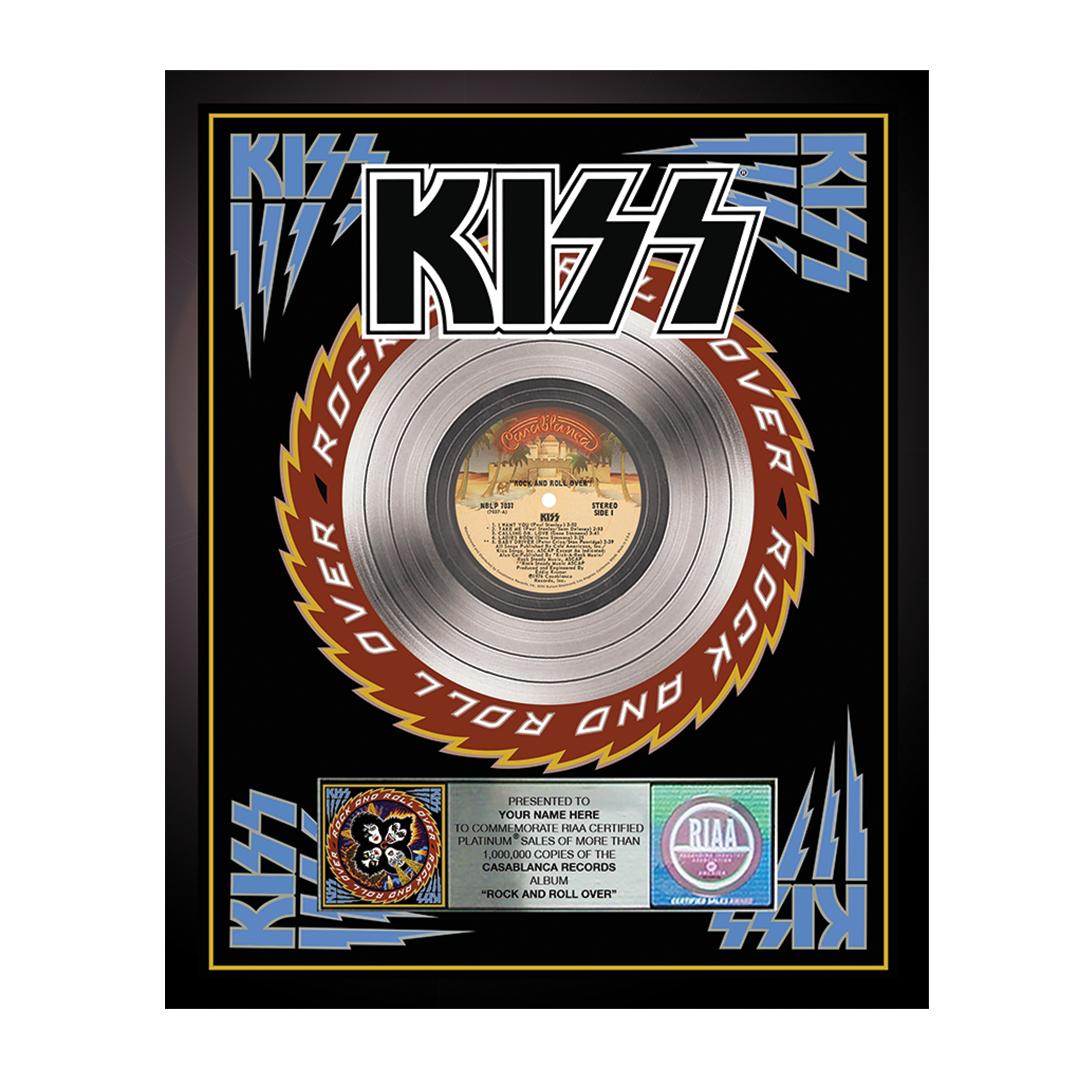The image depicts a commemorative platinum plaque for the band Kiss, awarded for selling over a million copies of their album "Rock and Roll Over" under Casablanca Records. The plaque features a black background and is encased in a stylish black frame, bordered by a thin gold line. Central to the plaque is a vinyl record with a striking platinum-silver finish, surrounded by a razor-bladed design akin to a chainsaw, accentuated with a red stripe. At the top of the plaque, the iconic Kiss logo is prominently displayed. The bottom section contains a customized banner reading "presented to your name here," alongside a picture of the band, marking it as an accolade for IAA-certified platinum sales.